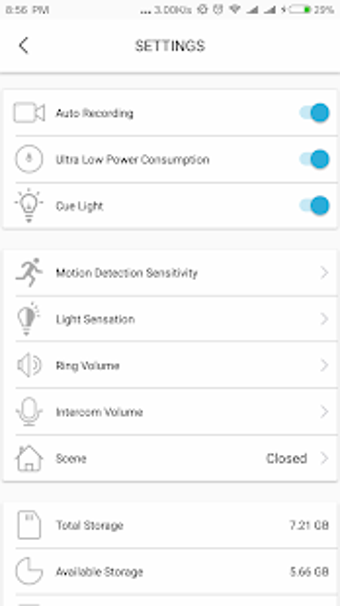The image displays a user interface with a light blue background. At the top of the screen, the status bar shows the time "8:56 p.m." and the available storage space "3.0 GB," along with a left-facing arrow icon and a settings gear icon. 

Below the status bar, there are three options, each outlined in blue boxes, accompanied by blue toggle switches:
1. **Auto Recording** – Toggle switch.
2. **Ultra Low Power Consumption** – Toggle switch.
3. **Cue Light** – Toggle switch.

Further down, there are five additional options outlined in blue boxes, each with a right-facing arrow indicating further settings can be accessed:
1. **Motion Detection Sensitivity**.
2. **Light Sensation**.
3. **Ring Volume**.
4. **Intercom Volume**.
5. **Scene** – Currently closed but can be expanded.

Finally, at the bottom of the interface, two more blue-outlined boxes provide storage information:
1. **Total Storage** – "7.21 GB."
2. **Available Storage** – "5.66 GB."

The concise layout of the interface ensures easy navigation and clear visibility of the device’s status and settings.